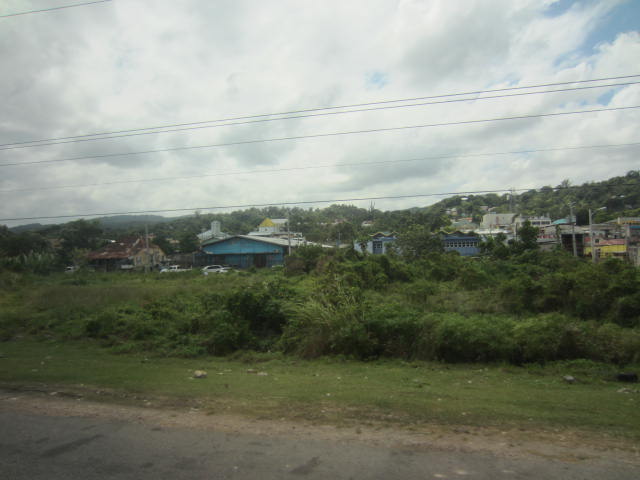This outdoor daytime photograph, rectangular and slightly wider than it is tall (approximately five inches wide by four inches tall), captures a rural landscape, possibly in an Asian country. The image prominently features a sky filled with white and gray clouds, with patches of blue peeking through, especially in the upper right corner. Power lines stretch horizontally across the midline of the photo, adding to the rustic charm. 

Below the clouds, a thin row of varied houses and structures extends across the image. These buildings include run-down shacks and vibrant blue and yellow homes with both sloped and flat roofs, some appearing slightly distant. There is also a larger building that resembles a hangar or warehouse towards the center-right.

The lower part of the photo reveals a simple paved road at the bottom edge. Adjacent to the road are patches of soil, short cut grass, rocks, and a mix of bushes, tall weeds, and other vegetation. To the left of the road, there's a run-down blue house with a shack beside it and white cars parked nearby. The scene includes a slight hill in the background, adding depth to the countryside setting.